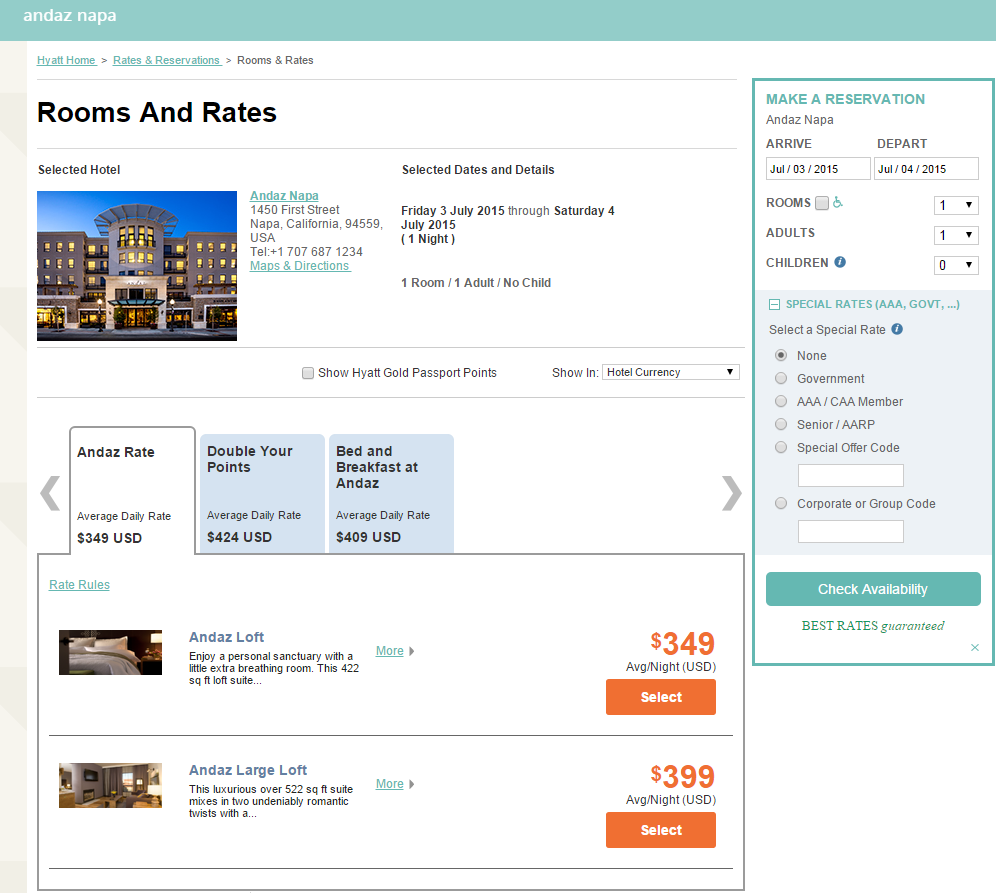**Detailed Caption:**

The image displays a hotel booking interface for Andaz Napa. The screen is front-facing and prominently features various room options available for reservation. Each room listing includes detailed information on the rates, types of rooms (such as standard rooms and suites), and pricing for different dates. The interface allows users to sort and filter options based on their arrival and departure dates, the number of adults and children, and any special rates or discounts available. The background is predominantly white, accented with subtle blue elements that add some vibrancy to the otherwise clean and professional design. The overall style of the booking site is functional yet slightly casual, offering a user-friendly experience for those looking to reserve a stay at Andaz Napa.